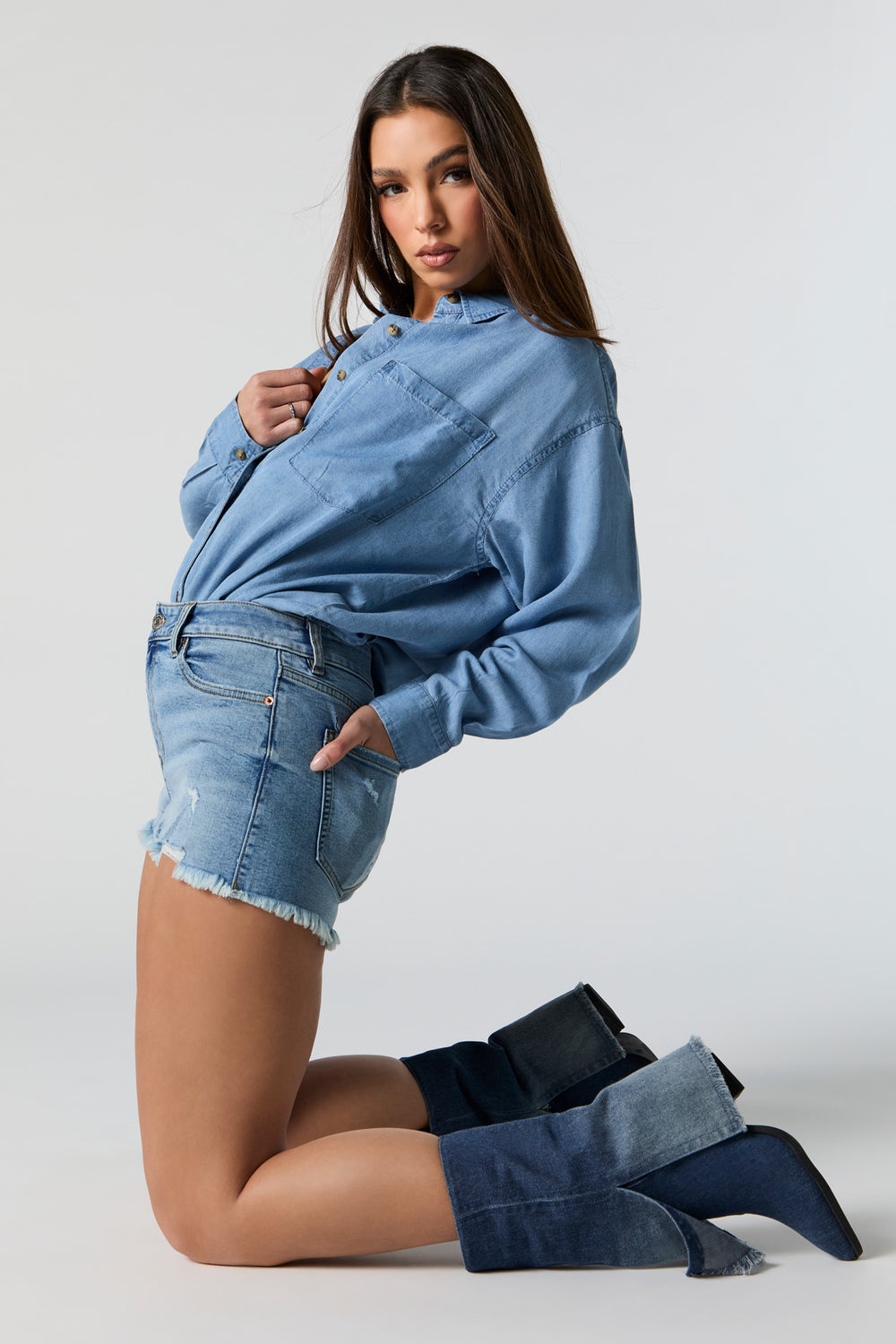In the image, a Caucasian woman is modeling clothing in a kneeling pose, facing the left but with her head and torso slightly turned towards the viewer, giving a seductive and engaging look. She has long, straight, dark brown hair and brown eyes, accentuated with neutral makeup. Her outfit consists of a white chambray long-sleeve button-down shirt, blue jean cut-off shorts, and blue denim boots that are folded down to calf-length but can reach up to her knees. Her right hand, adorned with a ring, is crossed over her chest while her left hand is tucked into her back pocket. The backdrop is a clean, featureless white with slight shadows, emphasizing the model without distraction.